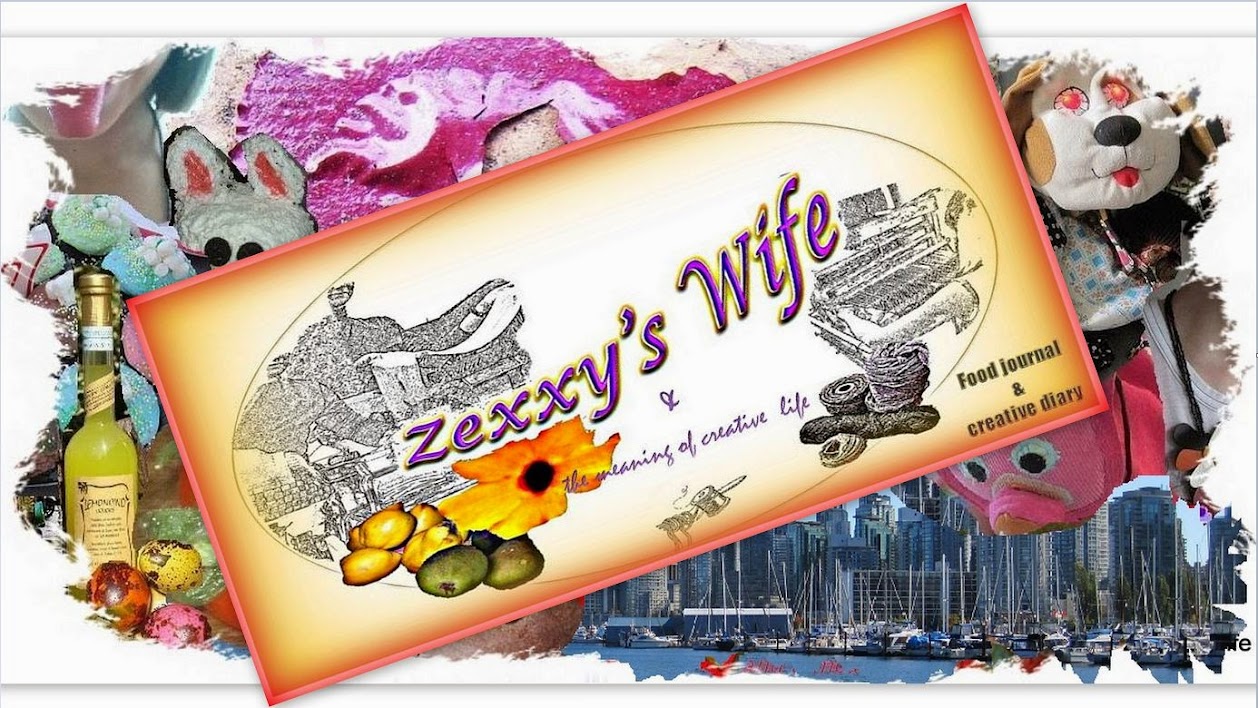The image is a complex, horizontal, rectangular collage that serves as an advertisement, featuring a layered and visually rich composition. The background is an abstract, colorful array reminiscent of a chaotic yet vibrant painting, interspersed with various objects and scenes. On the left side, there's a bottle of wine or liquor with a lime green liquid, accompanied by fruits and a tulip-like flower in gray. Above this is a stuffed animal that resembles a teddy bear.

On the right side, the background transitions into a city skyline during daytime, showcasing a harbor with docked sailboats and a distant view of skyscrapers. Among the skyline, some stuffed animals can be seen, including a pink figure that looks like a pig and a brown and white toy dog.

Superimposed on this vivid background is another diagonally placed rectangular image, rotated slightly counterclockwise. This rectangle features a gradient from dark tan to light tan towards the center and is bordered by a dark pink trim. Prominently displayed in purple, curved text are the words “Zexi’s Wife,” accompanied by the smaller, cursive subtitle “And the Meaning of Creative Life.” The lower right-hand corner of this shape indicates, in light black text, "Food Journal and Creative Diary."

On the left side of this overlaid rectangle, black and white illustrative images depict floral arrangements, fruits, and what appears to be a textile mill or statues, while the right side showcases a typewriter and pieces of yarn. The intricate layering and blend of imagery create a visually arresting advertisement that captures a multitude of elements, from creativity to everyday life.